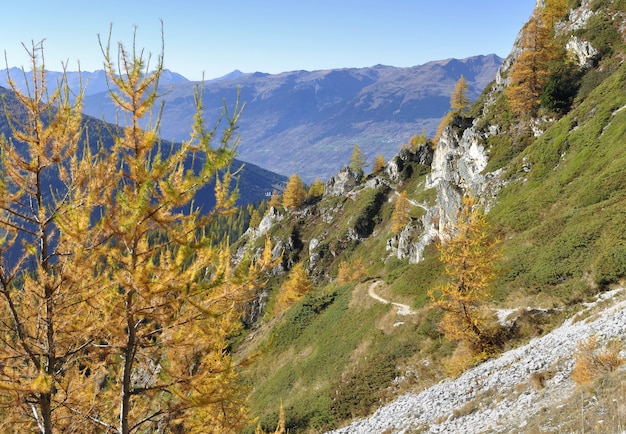The image is a detailed landscape photograph of a mountainous area taken on a clear, sunny day. On the right side of the horizontally rectangular frame, there's a green hillside with rocky outcrops and a noticeable path snaking along its surface. Central to the foreground stands a tree adorned with golden-orange leaves, suggesting the fall season. Additional trees with yellow and green leaves, alongside brown stems, dot the scene. Beyond the first mountain, there's another mountain range, leading to a large ridge of blue and grey hues in the background. The sky above is an expanse of clear blue, adding depth to the serene, natural environment. The photograph captures the tranquility of the landscape, inviting curiosity about the paths and the people who might traverse them.